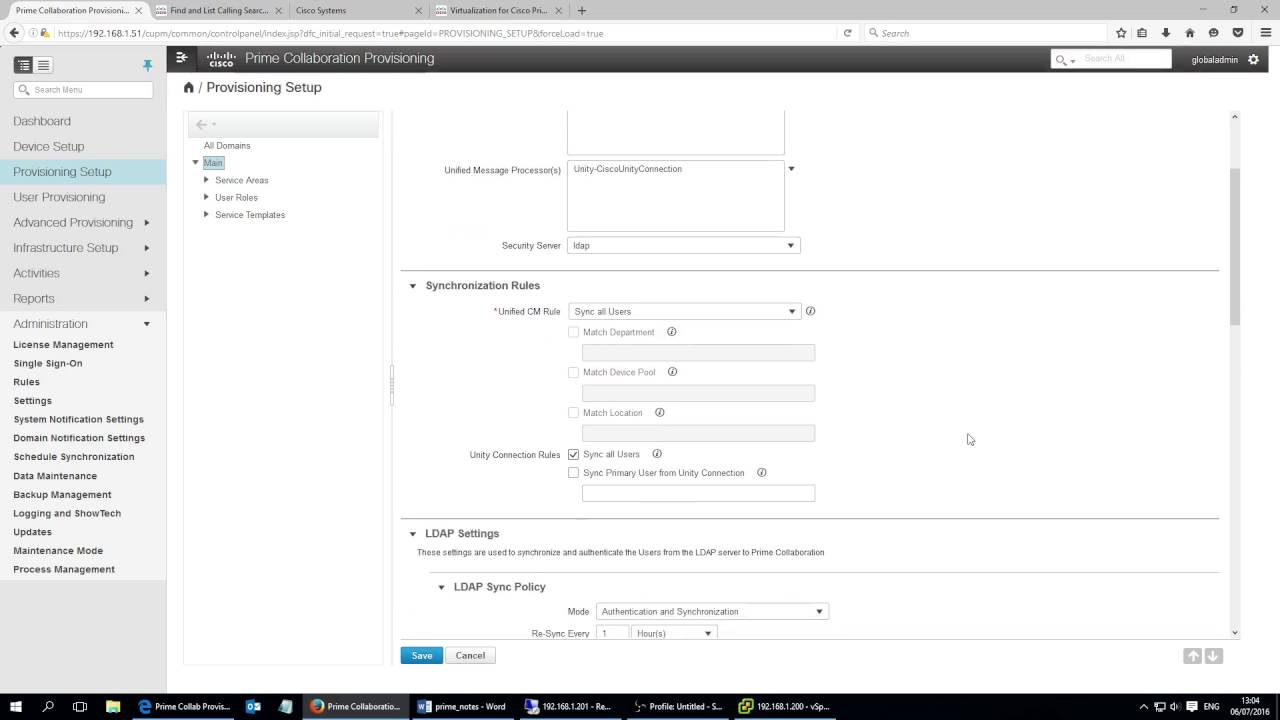This image showcases a computer screen displaying a web settings or setup page, potentially related to graphic design, programming, or a similar technical field. The photo, taken in landscape orientation, captures a detailed view of the page's layout and elements.

At the top of the page, a thin gray horizontal border features several pop-up tabs, with one tab prominently highlighted in a lighter gray color. The remaining tabs, though visible, have small, difficult-to-read text. Directly below this, a lighter gray bar includes a back arrow button, an address bar, and a search bar, followed by a series of icons allowing actions such as downloading, favoriting, returning home, and accessing a hamburger menu.

On the left side, there's a vertical sidebar structured in a column format, offering various options such as Dashboard, Device Setup, and Provision Setup. The Provision Setup option is selected, indicated by a blue border.

Adjacent to this sidebar, another vertical section titled "Provisioning Setup" presents multiple options for selection. To the right, a prominent white area titled "Synchronization Rules" contains several customizable drop-down boxes.

Below the Synchronization Rules section, there's an area dedicated to LDAP settings. At the bottom of the page, two buttons are visible: a blue 'Save' button and a 'Cancel' button, providing options to either save the changes or cancel the operation.